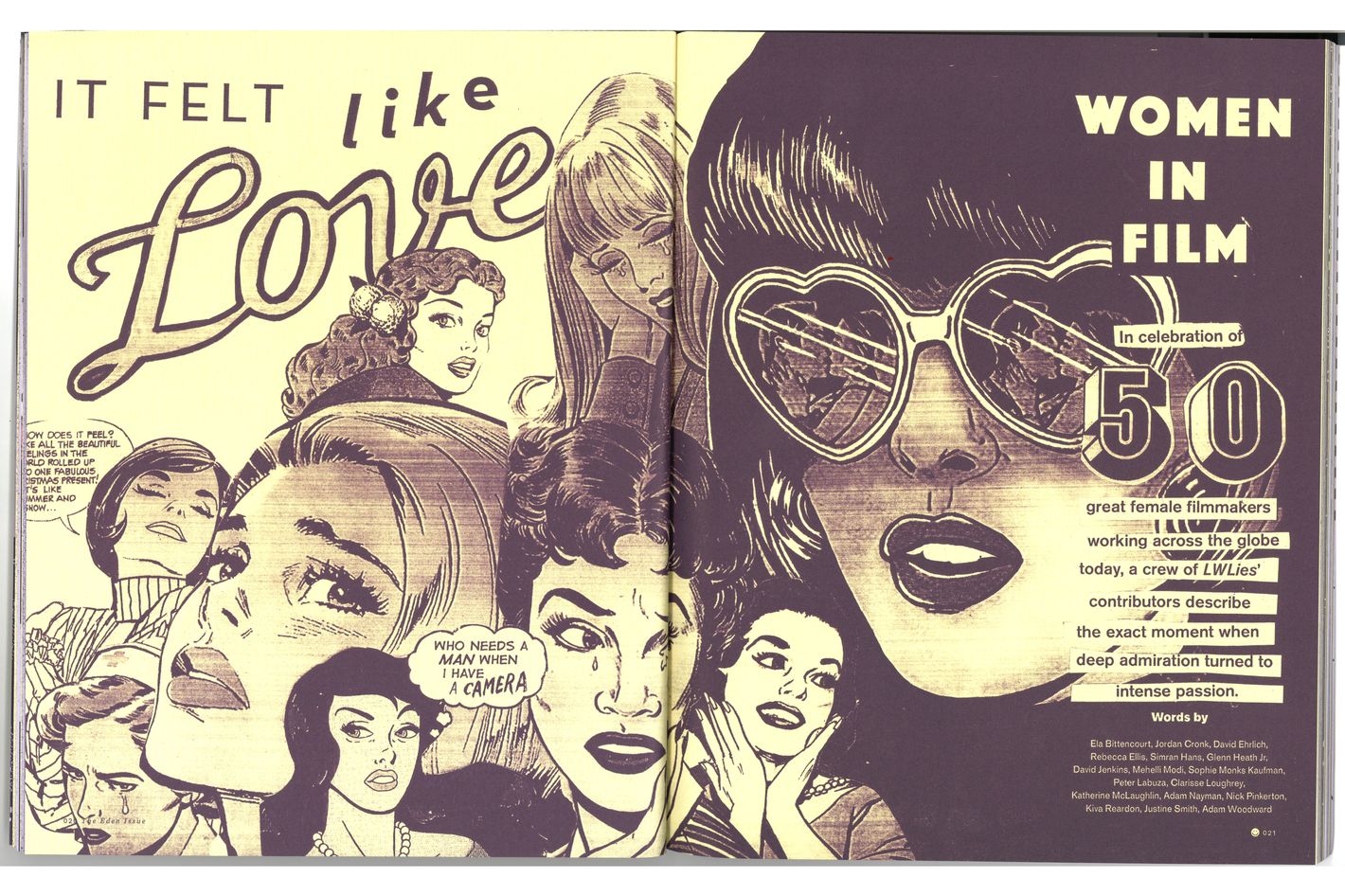The image is a detailed cartoon illustration spread across two pages of an open book, with a dark green hardcover. The artwork appears to be an artist’s rendition in a blend of black, yellow, and an old-school photograph style with a red hue. The pages feature headshots of various women, styled similarly to a comic book. These women's faces are designed with a vintage artistic approach, showing diverse expressions and poses.

On the left page, the heading reads, "It Felt Like Love," while on the right page, the title states, "Women in Film: In Celebration of 50 Great Female Filmmakers Working Across the Globe Today." This title emphasizes an homage to pioneering women in filmmaking. The text describes contributions from LW Live's contributors detailing moments when admiration turned into intense passion for film.

Among the distinctive illustrations, one woman, located prominently on the right-hand side, is depicted wearing heart-shaped sunglasses with visible reflections of a man and woman kissing. She has black hair, wears red lipstick, and her face is notably darker in hue. Beside her, another female figure smiles while holding her face in her hands. Additional headshots include a woman with tears streaming down her face, a lady peering upward as if about to cry, and others adorned with varying hairstyles and makeup. One of the women is portrayed with flowers in her hair. The composition includes text bubbles accompanying each face, one of which reads, "Who Needs a Man When I Have a Camera?"

The overall color scheme maintains a subdued palette, integrating black, yellow, and variants of red and brown, lending the illustration an almost grayscale, nostalgic feel. The detailed and expressive portrayals of women throughout the spread capture a celebratory and introspective look at female filmmakers and their journeys.